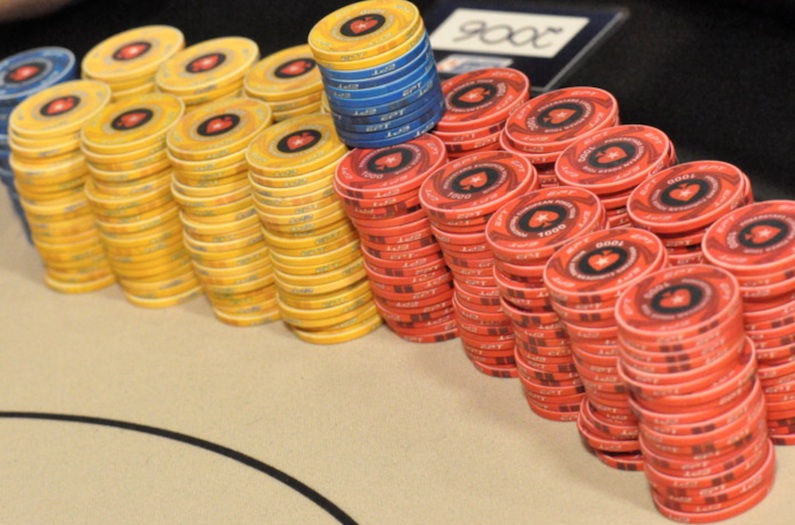This photograph, taken indoors in landscape orientation, showcases an up-close view of various poker chips organized in a curved alignment on a table. On the right side, there are ten stacks of reddish-orange poker chips, each stack containing approximately 20 chips. These chips feature a white trim, a black inner circle with a red spade and star design, and a denomination of 1,000 in white. To the left of these, there are eight stacks of yellow poker chips that share the same black circle and red spade design, though their denomination is obscured due to the image’s blurred quality. Further left, there is a single stack of blue poker chips, also with the red spade in the black circle, but the value remains unreadable. Atop the eight reddish-orange chip stacks, there is a shorter pile of blue chips with two yellow chips placed on top. The table appears off-white with a black line running through it. In the background, beyond the chips, a white rectangular object bearing the upside-down number "2006" can be faintly seen.